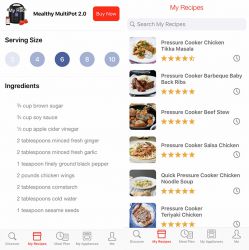This image appears to be a screenshot from a recipe app displayed on a smartphone. The header reads "Monthly Multi-Port 2.0." Below this, there is a red box containing text that is not legible due to the image's small size. On the right side of the screen, beneath the header, it says "My Recipes" followed by a search bar. Further down, the app displays six recipes, each accompanied by an image of the corresponding dish. The recipes listed are:

1. Pressure Cooker Chicken Tikka Masala
2. Pressure Cooker Barbecue Baby Back Ribs
3. Pressure Cooker Beef Stew
4. Pressure Cooker Salsa Chicken
5. Quick Pressure Cooker Chicken Noodle Soup
6. Pressure Cooker Teriyaki Chicken

On the left side of the screen, there is a serving size indicator with options for 2, 4, 6, 8, and 10 servings. The indicator is set to 6 servings. Below this section, there is a bolded "Ingredients" label with a list of ingredients written faintly underneath.